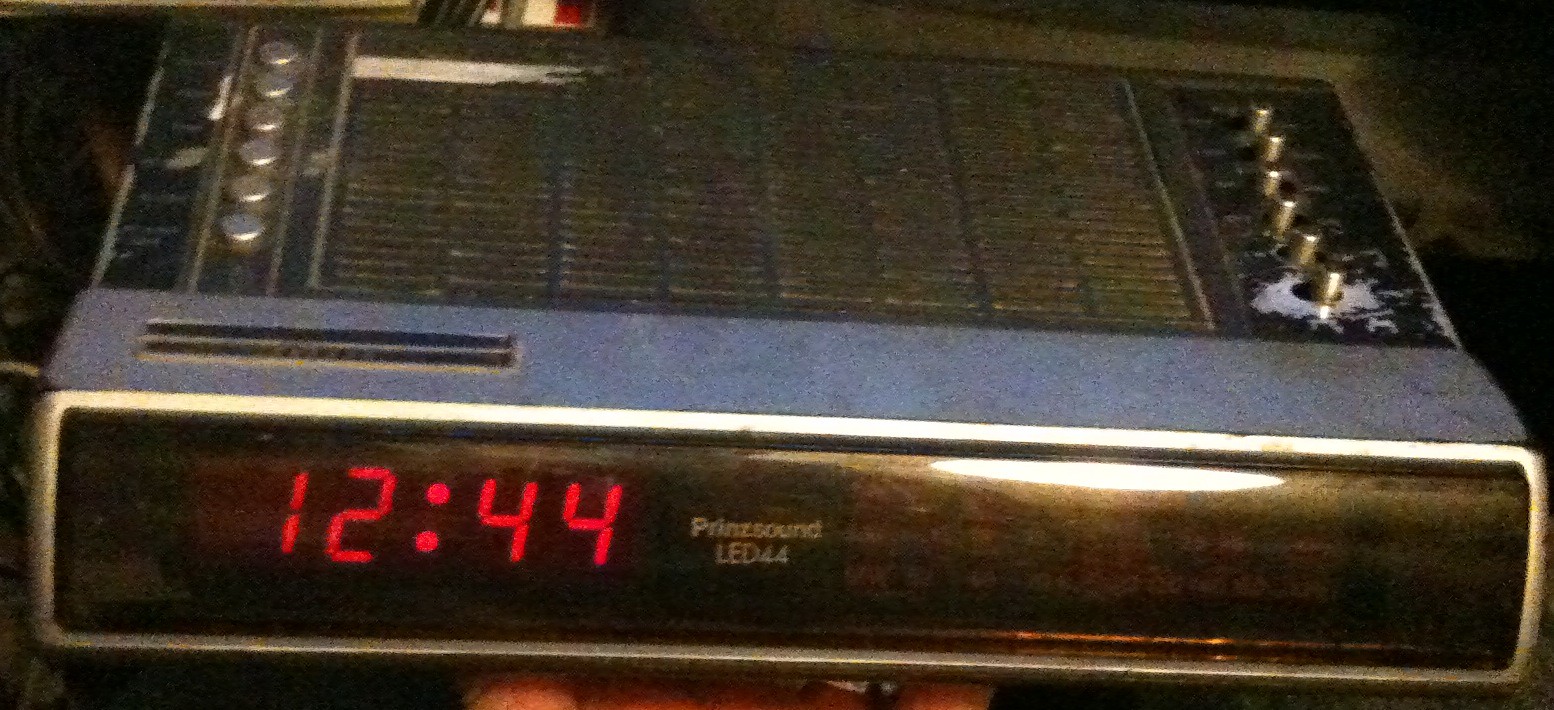This photograph captures a vintage alarm clock likely from the late 90s or early 2000s. The clock is rectangular in shape, with a longer width than height, and features a blend of silver and black surfaces. Dominating the black front panel is a red LED display showing the time "12:44," with the logo "Prinsound LED 44" placed in white text to its right. The front panel appears to be covered with a glass or plastic pane. Above the display and logo, silver flat spherical buttons are aligned on the left side, contrasting with knob-like buttons on the right. Centrally on the top surface, there are visible grates, possibly part of a vent system, showing signs of dirt and browning. The background suggests the clock is placed in a somewhat cluttered, dimly lit room. At the bottom of the photo, a hint of an orange object and a light-skinned hand holding up the clock can also be seen.